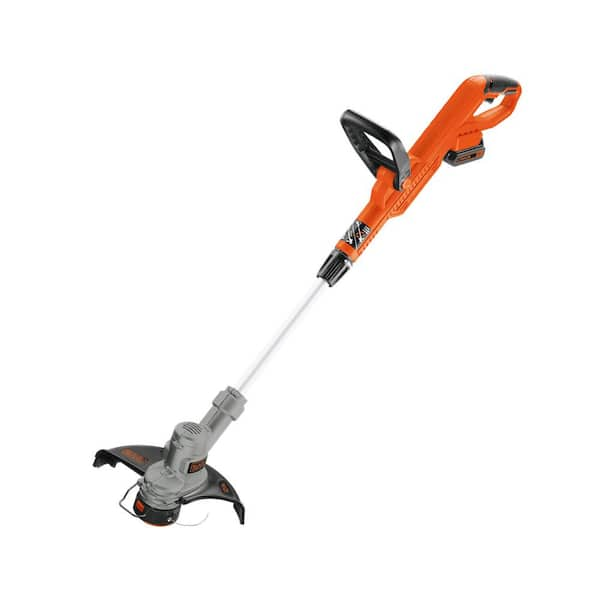This photograph showcases a cordless electric weed whacker set against a completely white background. The top section features an ergonomic handle, predominantly orange in color, interspersed with black elements, including a small push button. Directly beneath the handle is a black component resembling a battery pack. Further down, attached to the middle section, is an additional handle, also black, for better grip and maneuverability. Connecting the handles to the operational end is a silver metallic shaft. At the bottom of the tool, there's a cylindrical gray housing encasing the motor and spinning blades, protected by a black shield. The cutting head, equipped with multiple strings, culminates in a black segment with a red button for string release. The image emphasizes the tool's sleek design, portability, and battery-driven convenience.